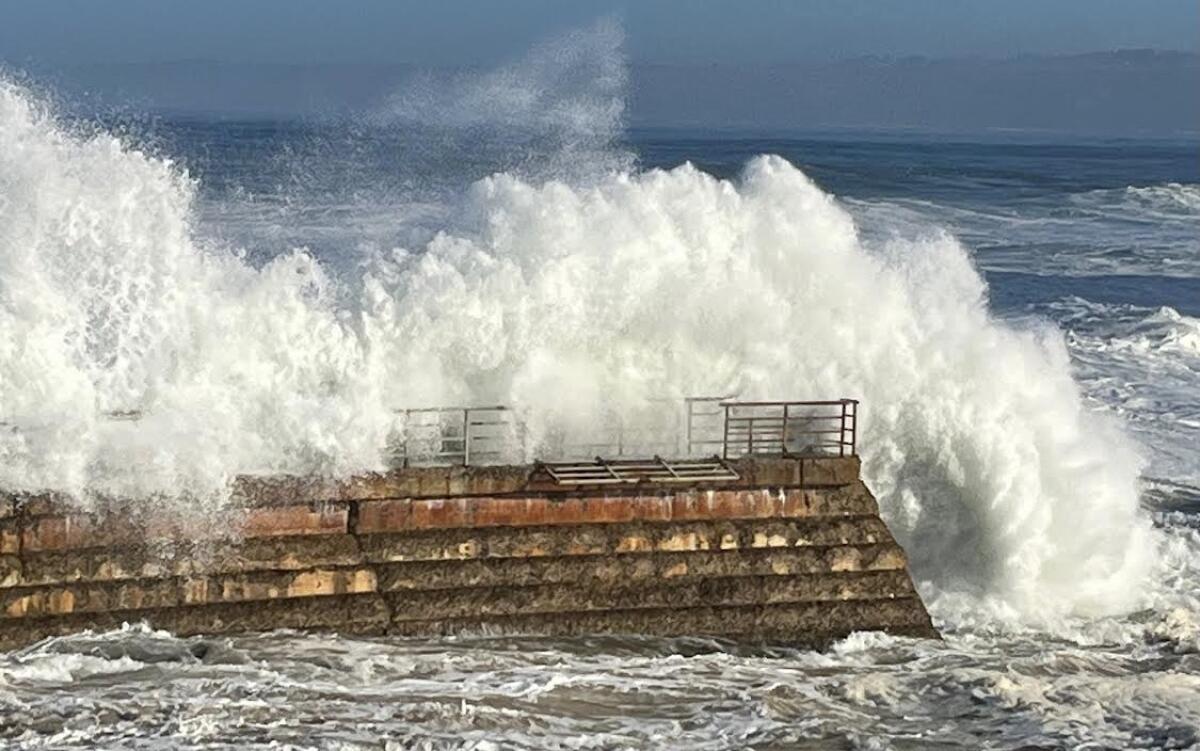In this striking image, towering waves crash with immense force against a cement and steel barrier reef that resembles a stepped jetty extending into the turbulent ocean. The waves, crowned with white caps, surge dramatically, creating an atmosphere of raw and powerful energy. The walkway along the jetty, adorned with handrails, reveals signs of damage, with sections of the railing toppled over by the relentless assault of the sea. Despite the ferocity of the waves, the ocean beyond remains visible, though equally restless, painted in hues of deep blue under the churning skies. The backdrop features a contrasting landscape, with a mountain range peeking through under a gloomy, grey sky, adding a sense of depth and scale to the scene. This photograph beautifully captures the dynamic interplay between man-made structures and the relentless forces of nature.